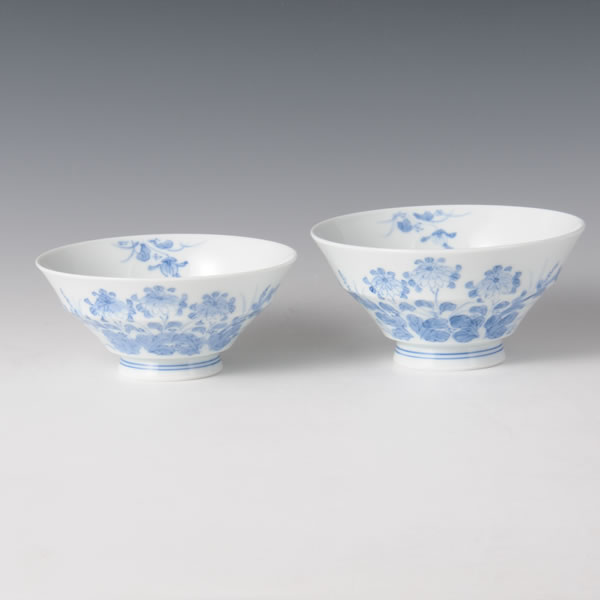The image is a close-up photograph of two white china bowls adorned with royal blue floral designs. The bowl on the left is slightly smaller than the one on the right. Both bowls feature delicate blue flowers, with three prominently displayed on their exteriors and additional floral motifs decorating their interiors. The bowls, which could be made of glass or ceramic, have a small blue stripe along their thin bases. They are set against a gray background, which transitions from darker at the top to lighter at the bottom, enhancing the elegant contrast of the blue and white designs.